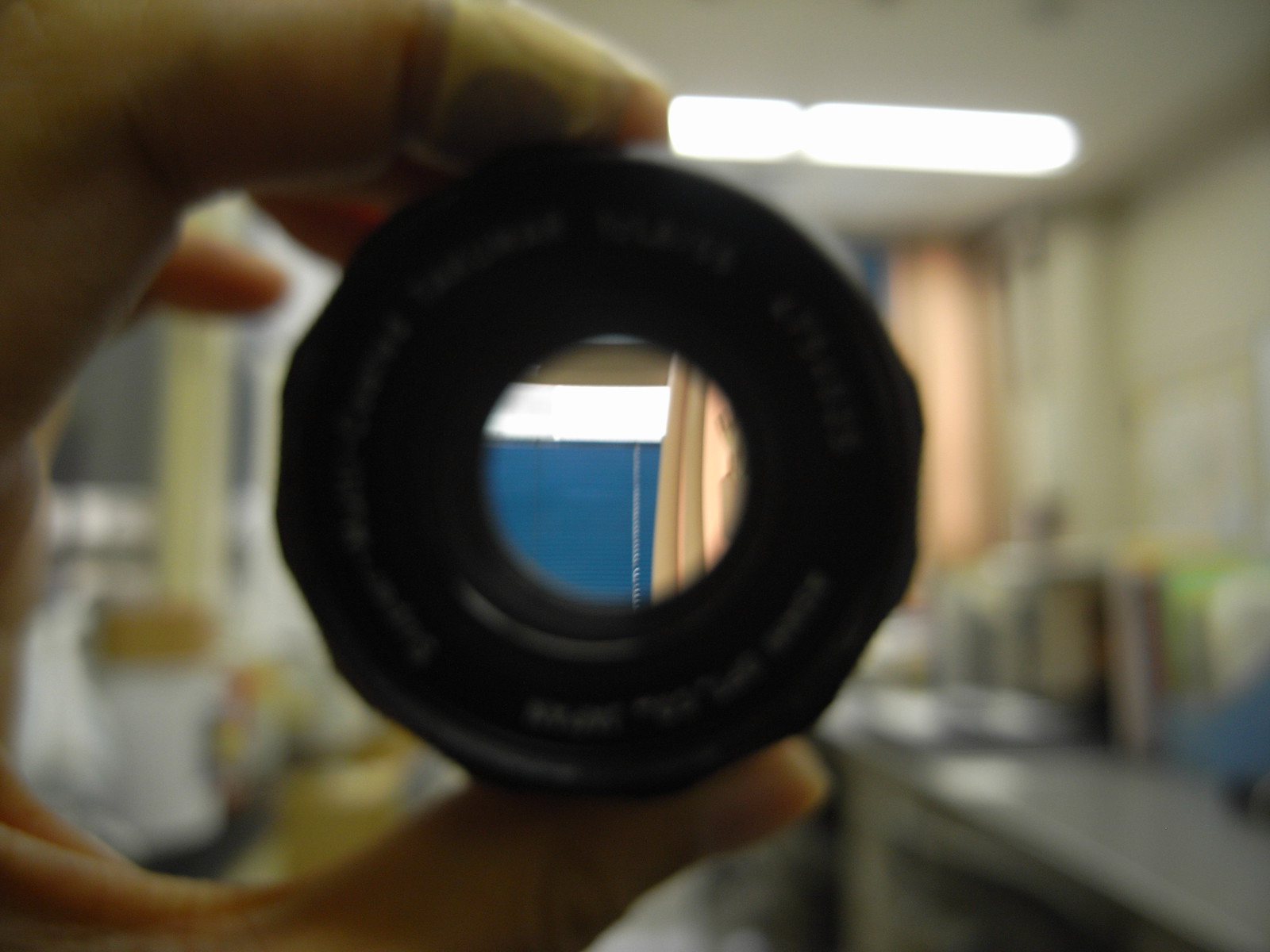The image features a hand prominently positioned on the left side, with an index finger wrapped in a bandaid, holding what appears to be a dark toy truck tire or a small ring, approximately 3 inches in diameter. The bandage on the finger and the grainy texture of the tire, possibly rubber with white lettering, stand out. The backdrop through the ring reveals a somewhat blurry interior scene with a distinctive blue background, complemented by a yellow curtain. The setting appears to be either a kitchen or a lab/workshop, indicated by countertops on both sides and various bottles and books scattered around. A ceiling light is visible above, and the overall environment is filled with indistinct shapes, suggesting a cluttered workspace.